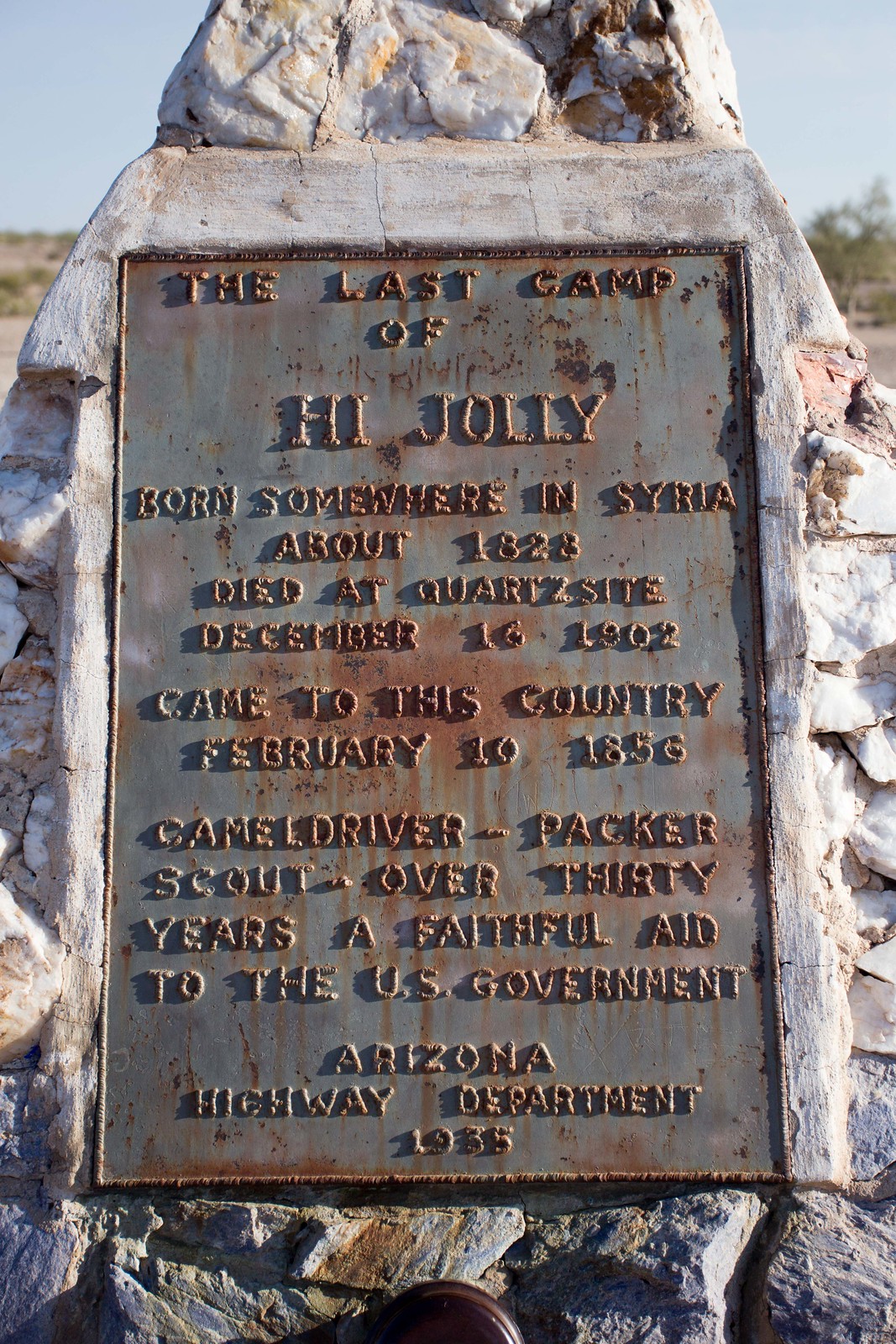The image displays a close-up of a large, irregularly-shaped white rock with a bronze plaque that has oxidized, giving it green and brown hues. The plaque is dedicated to High Jolly and reads: "The last camp of High Jolly, born somewhere in Syria around 1823, died at Quartzsite, December 16, 1902. Came to this country February 10, 1856. He was a camel driver, packer, and scout, providing over 30 years of faithful aid to the U.S. government." The plaque also notes that it was erected by the Arizona Highway Department. While the precise date of dedication is under debate, it is mentioned to be either 1935, 1955, or 1966.